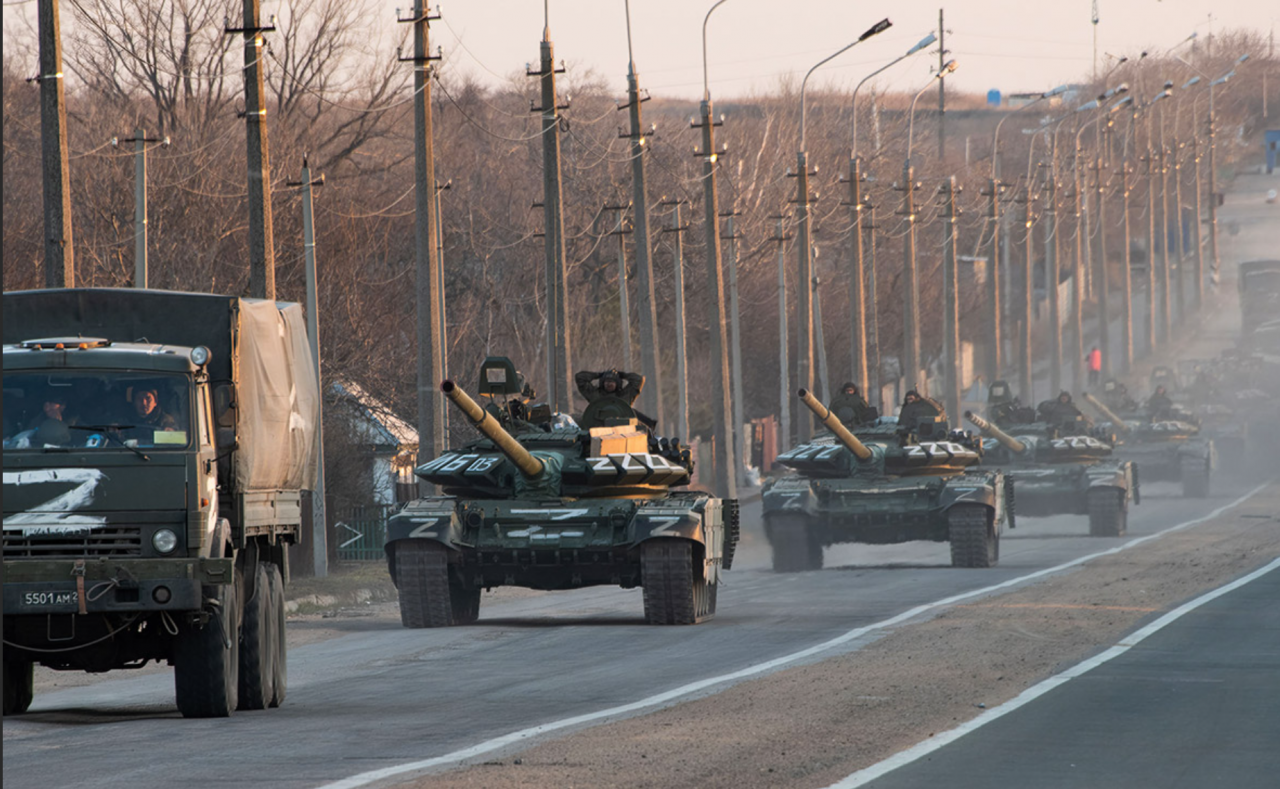The photograph captures a daytime scene of a warzone, showcasing a military convoy advancing down a dusty road. The convoy, consisting of four low-riding, dark green tanks and a large transport truck with a covered back, is moving from the center right of the image towards the lower left-hand corner. Each tank and the truck prominently feature a white letter "Z" painted on their fronts. The tanks, with their firing barrels elevated, have two soldiers each—one manning the cannon and the other scanning the surroundings. The transport truck also contains two men. The road, marked with white outlines and a central median of brown dirt, is flanked by tall telephone poles and leafless trees. Dust clouds rise from the vehicles' movement, partially obscuring the background and adding to the gritty atmosphere of the scene.